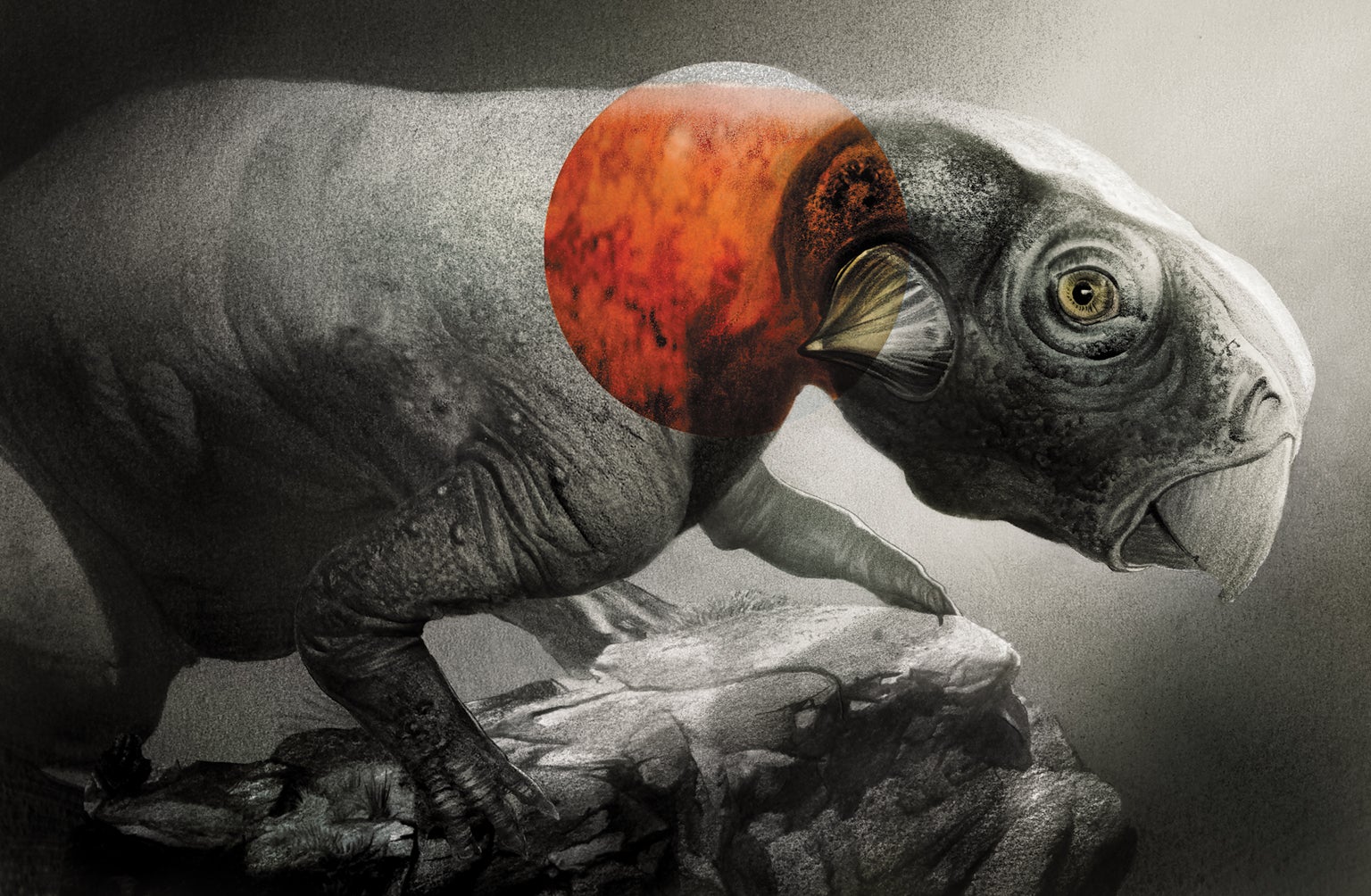This image showcases a detailed close-up of a fantastical creature that seems to blend elements of various animals and prehistoric beings. Predominantly in black and white, it features subtle yet significant color accents—a light red circle highlighting the area around the creature's neck and a soft amber eye with a blue pupil. The creature's head has dragon-like, reptilian qualities with a beak reminiscent of a turtle's, and points that may resemble ears or horns. Its powerful, hairless body has a texture similar to elephant skin, seated firmly on a rocky surface under varying shades of gray light. The background shifts from gray to white, creating an ethereal, almost otherworldly atmosphere. Four legs are visible, the front appearing worm-like, hooved, or arm-like, while the hind legs seem more robust, supporting the creature's stance on this illuminated, textured rock. The precise nature of the creature remains ambiguous, blurring the lines between a fantastical, prehistoric, or even microscopic entity.